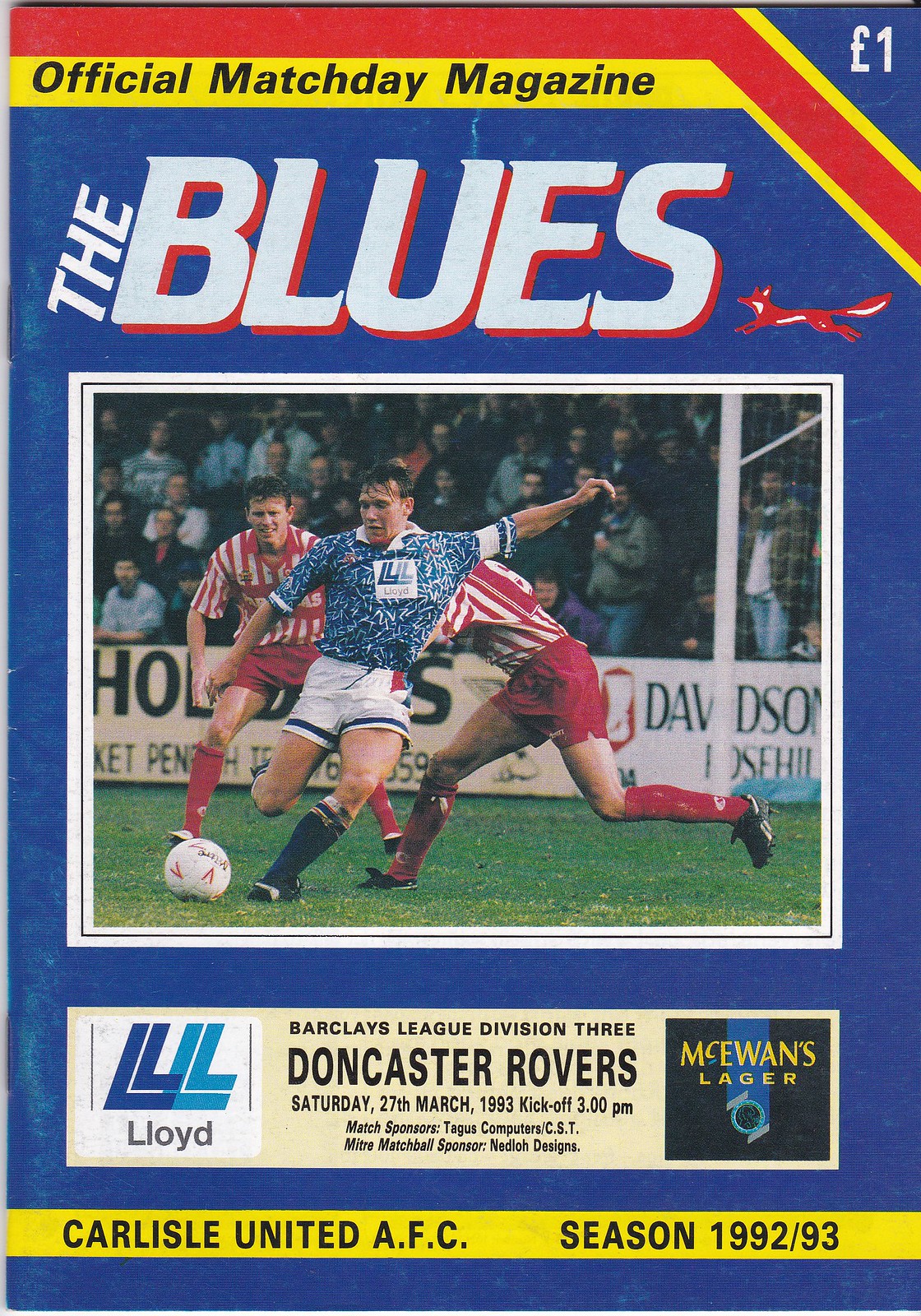The cover of the British football match day magazine, titled "Official Match Day Magazine," features a vivid design with blue as the primary color, complemented by red and yellow accents, and white text. The top right corner displays the price "one British pound" in a yellow bordered box with black text. Prominently, the title "The Blues" is written in white, accompanied by an illustration of a fox. Below, a dynamic scene depicts three soccer players on a field: one in a blue shirt with white accents, blue shorts and socks, kicking a white ball, while two opponents in red and white striped shirts, red shorts, and red socks, try to intercept him. At the bottom, it reads "Barclays League Division III Doncaster Rovers, Saturday, 27th of March, 1993, kickoff 3 p.m.," followed by sponsor names including "McOwen's Lager" and "Lloyd." Finally, a yellow stripe at the base of the cover declares "Carlisle United AFC Season 1992-93."